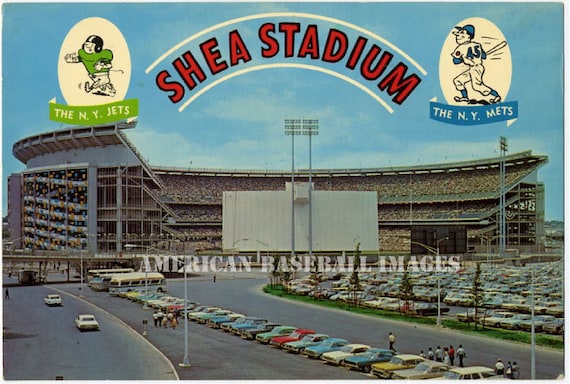This image is a vintage, color photograph of Shea Stadium, appearing as though it could be a postcard from the 1960s. At the top, bold red letters arch the stadium name, "Shea Stadium." On the left side of the photograph, there's a small cartoon logo featuring a football player captioned "New York Jets," and on the right side, an image of a baseball player labeled "New York Mets." The photo, marked with a watermark stating "American Baseball Images," shows a packed stadium, suggesting an ongoing game, and a bustling parking lot filled with old-style cars from the 1950s and 1960s. The sky in the background is blue with a few small clouds, further accentuating the nostalgic, bustling energy captured in this vintage image.